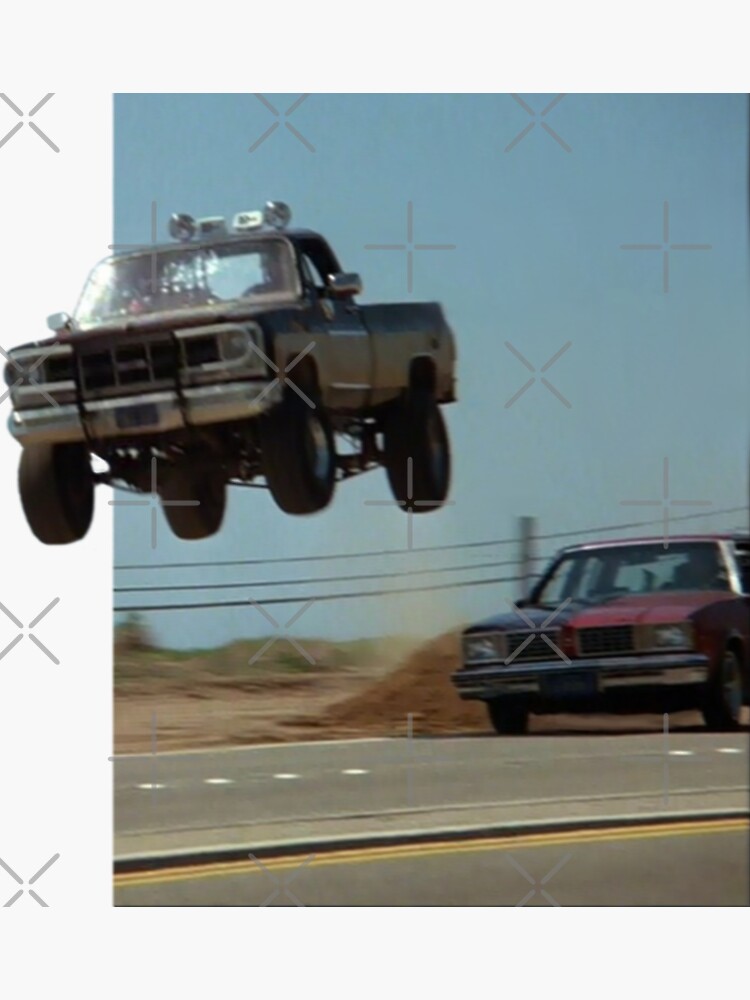This vividly surreal and dynamic image captures an intense action scene resembling a movie stunt. The focal point is a heavily modified, dark-colored pickup truck, mid-air, as if it just launched off a ramp. This truck, reminiscent of a Mad Max vehicle, features thick tires, a reinforced silver bumper, and large chrome spotlights atop its roof. Its paint is a striking combination of metallic brown and darker hues. Visible within the airborne pickup is a shadowy driver outline.

Below and behind the pickup, a two-toned car—red on one side and blue on the other—appears to be in pursuit. This car, possibly a police vehicle, is driving along a gray paved road with white dashed lines and a double yellow centerline. Adding to the surreal quality, elements throughout the image, such as X's and cross-hatches, suggest digital alterations.

The background shows a clear blue sky above a desert landscape, with blurred utility poles stretching horizontally and hints of green vegetation amid the dusty, brown terrain. The scene exudes a sense of high-speed chaos and cinematic drama.